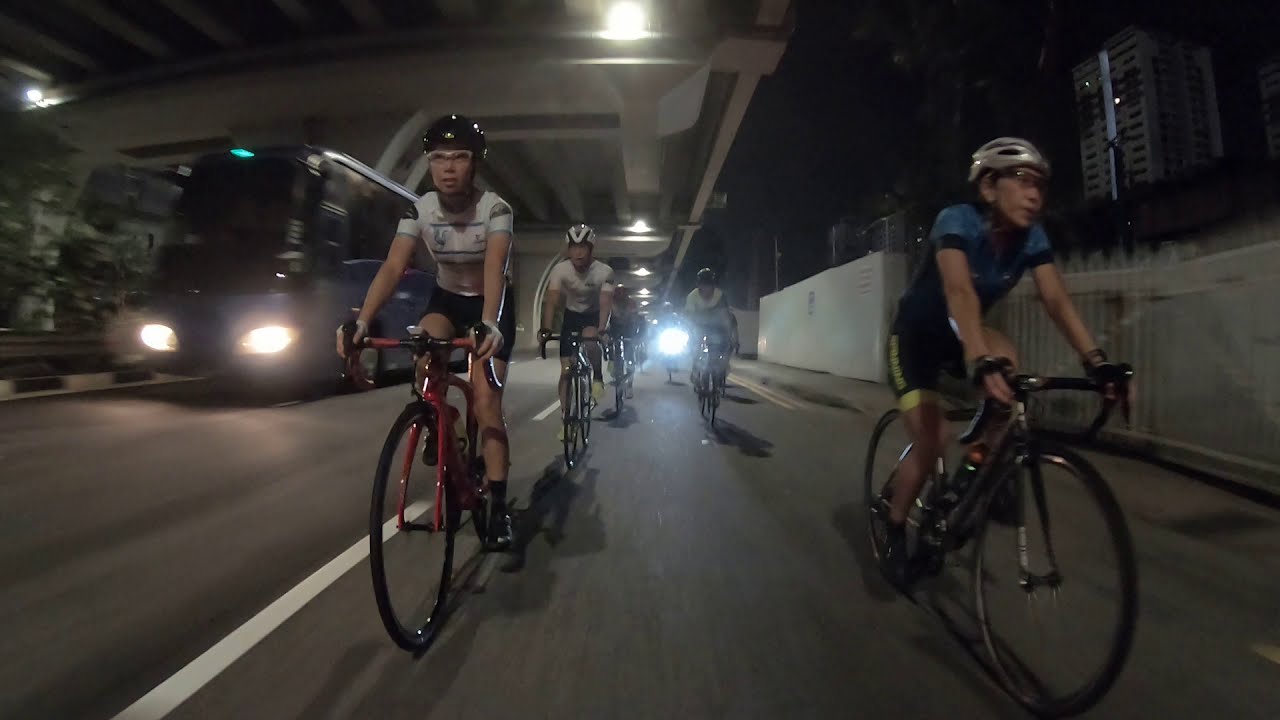In this horizontal, rectangular image, a group of male bicyclists, clad in tight-fitting shorts and a variety of colored t-shirts, navigate a bike lane at night. They are all wearing helmets and glasses, adding a layer of safety as they ride in a row along the side of the road. The scene is cast in darkness, with the only illumination coming from roadside lights, the overhead lights of an overpass, and the lights of a large blue bus to the left. The bus, a black and silver double-decker, is driving in an adjacent traffic lane with its interior lights off, making it appear blackened out. In the background, some tall buildings are faintly visible against the dark sky, adding depth to the urban night scene. A cement area marks the end of the road on the right side, and beyond it, there's a hint of grass, suggesting a park or open space. One of the bicycles far in the distance might have a light, but the riders in the foreground do not, further emphasizing the nocturnal setting.